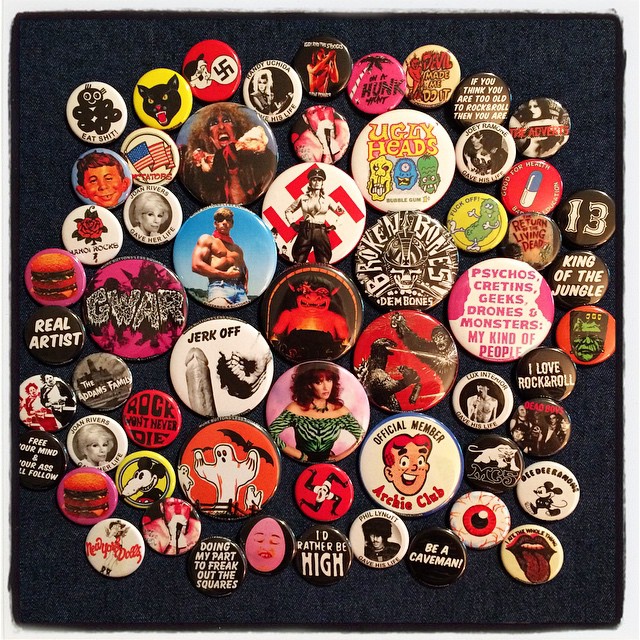The image showcases a vibrant, eclectic collection of approximately 40 to 60 button badges spread across a dark, possibly dark blue or gray, fabric background. The buttons, primarily adorned with diverse and colorful designs, feature various inscriptions and images that reflect an array of interests and themes. Central to the collection are larger buttons, encircled by smaller ones around the perimeter. Among the notable buttons, there are some with comic characters like Archie from Archie Comics, one with Peg Bundy on a pink background, and another featuring a ghost. Some buttons come with provocative inscriptions such as "I'd rather be high," "Be a caveman," "Doing my part to freak out the squares," "Free your mind, your ass will follow," and "Real artists, psychos, geeks, drones, monsters, my kind of people." Others simply display numbers like 1 and 13 or symbols, including swastikas. The collection reveals a juxtaposition of whimsical and controversial icons, suggesting it might be part of an individual's diverse and personal assemblage. Mixed in with the text are images of animals—cats, dogs—and a muscular man, adding to the eclectic visual narrative of the buttons. The badges are a mix of vibrant red, black, white, blue, yellow colors, each contributing to the overall patchwork of this unique display.